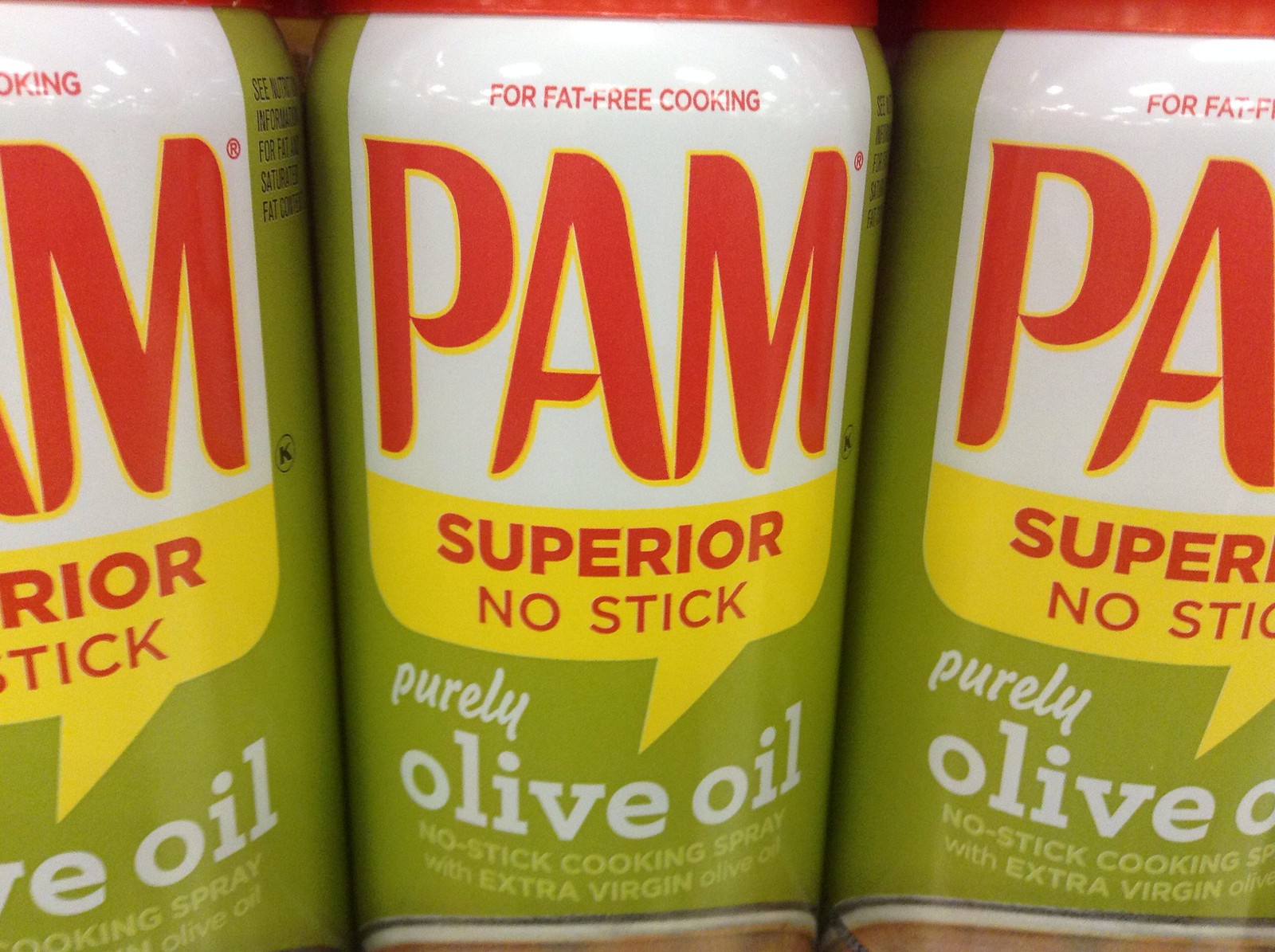Three green spray bottles of PAM cooking spray sit neatly on a shelf. The bottles are designed in an olive green hue, reminiscent of fresh olives, aligning perfectly with their content. The word "PAM" is prominently displayed in large red letters, outlined with yellow, all set against a clean white background. Just below, in smaller red text against a yellow backdrop, are the words "Superior No Stick." The phrase "Purely Olive Oil, No Stick Cooking Spray with Extra Virgin Olive Oil" is written further down in white text. At the top of the bottle, an additional claim states "For Fat-Free Cooking." The trio of spray bottles stands orderly, ready for use in any kitchen seeking a healthy, fat-free cooking solution.